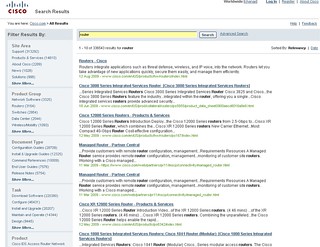A screenshot of an archaic-looking Cisco web page, characterized by its blurry and dated design. The page prominently displays the search results section, indicating that a query has been entered, as evidenced by the highlighted yellow search bar containing text. Seven distinct search results are visible, though more likely exist beyond the visible portion of the screen. The web page offers filtering options, situated in five discrete boxes containing links, which are, unfortunately, illegible due to the blurriness. The overall appearance and functionality suggest an early version of web design, reflecting Cisco's technological interface from a bygone era.